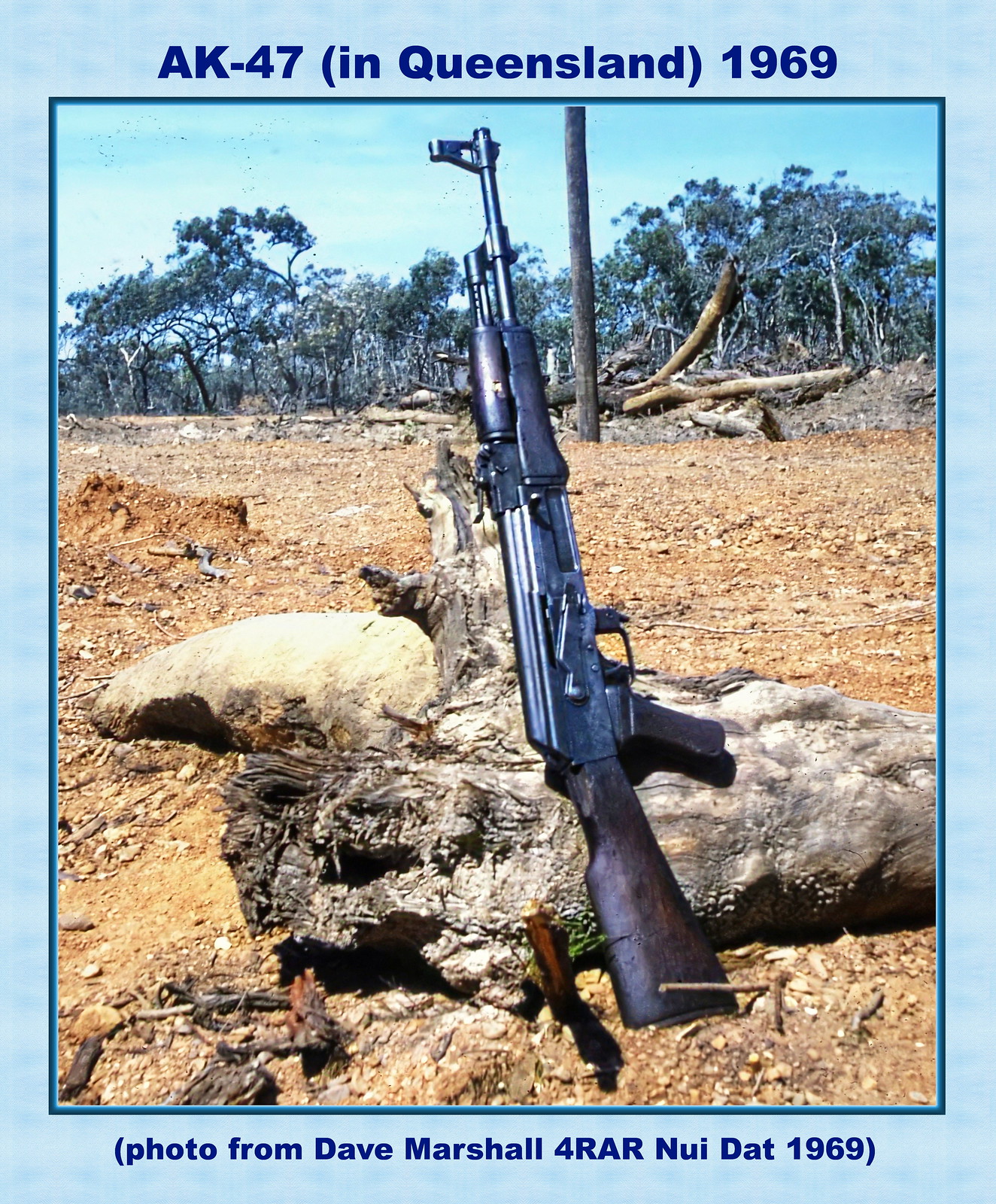This vintage photograph, taken in Queensland in 1969, depicts an AK-47 automatic rifle leaning vertically against a large, flat-topped rock on a desolate beach with a brown, gravelly dirt ground. The rifle, primarily black with a dark wooden stock, is positioned so that the barrel points upwards to the sky while the butt rests slightly to the right of the rock's base. To the left of the rifle, another lighter tan rock is visible. The background features a small section of forest or jungle, with scattered rocks and a fallen tree, adding to the rugged and historical atmosphere. The sky above is a clear blue. A caption at the top reads, "AK-47 in Queensland, 1969," and below the photo, it states, "Photo from Dave Marshall, 4RAR Nui Dat, 1969." The photograph, though somewhat faded and soft in resolution, vividly reflects its Vietnam War era origins.